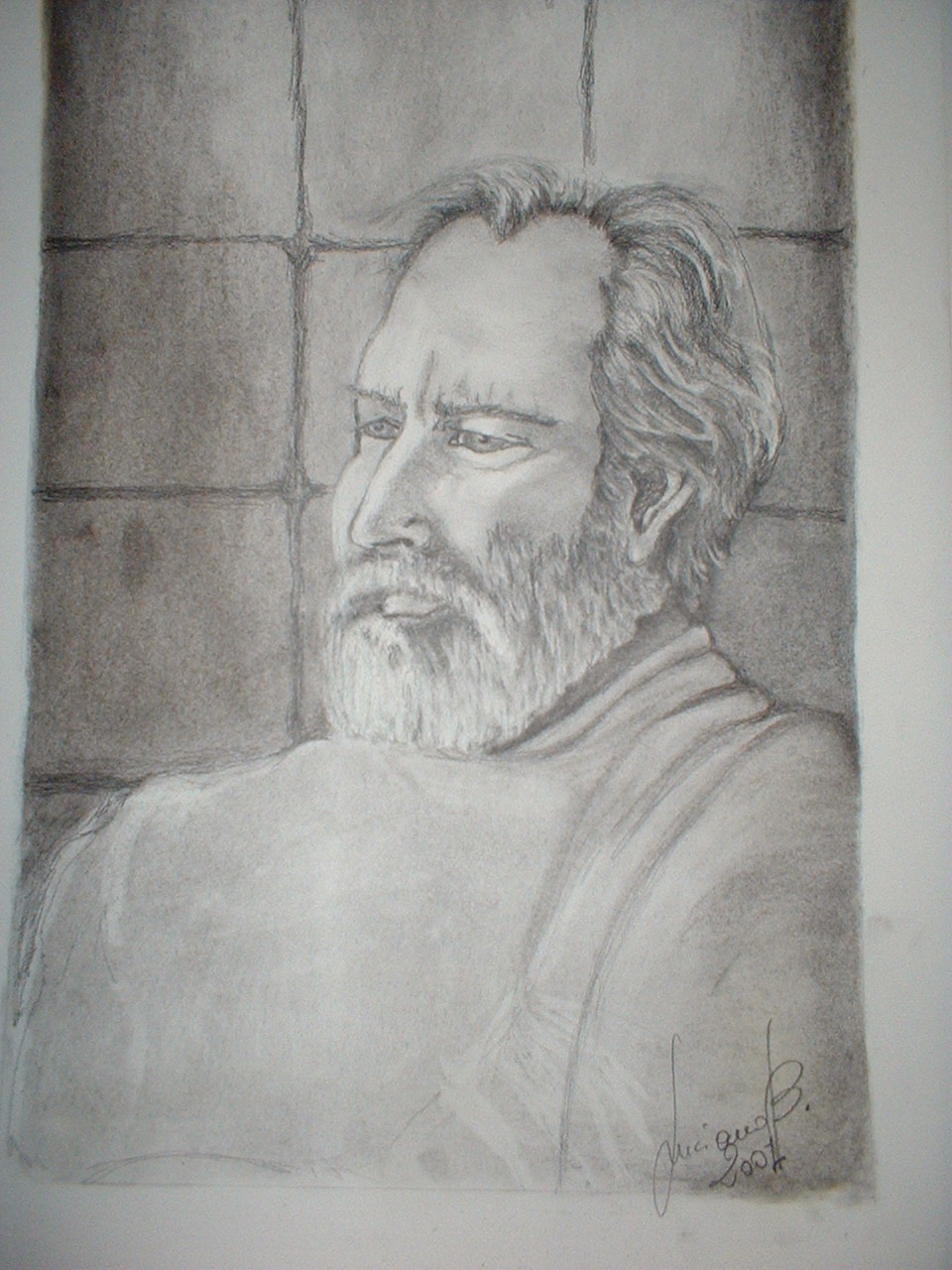This image showcases a meticulously detailed pencil drawing of a man, set against a greyish background that resembles a tiled wall. The man, who has a heart-shaped face with short, shaggy whitish hair, a full beard, and a moustache, is gazing seriously off to the left. His expressive face features furrowed brows and greyish eyes. He appears to be wearing a pale, possibly white top, but the garment has an unusual square-like shape around the chest area that doesn't align perfectly with the rest of the top. Atop the intricately drawn background, there's a white outline framing the image. In the bottom right corner, the artist's signature is visible in cursive handwriting, accompanied by a number that appears to be from the year 2001, although the signature itself is not entirely legible.